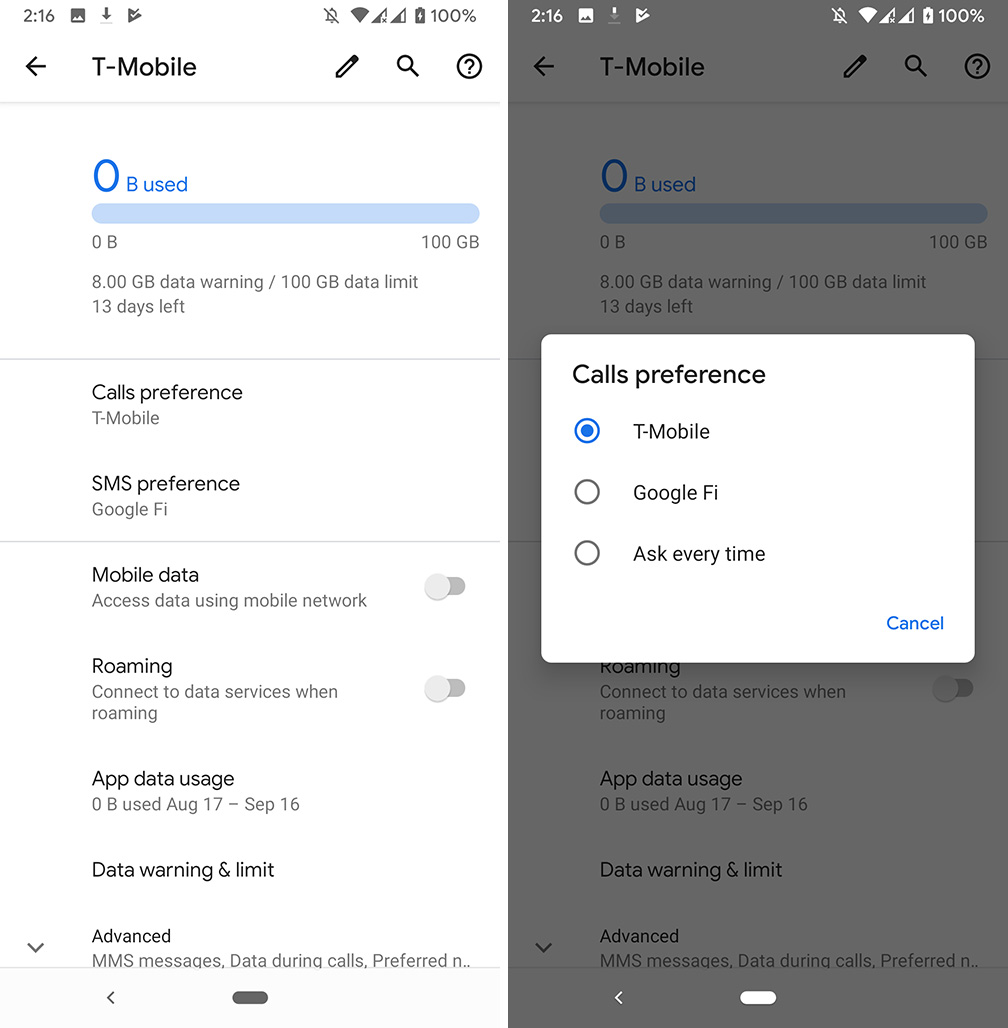This pair of sequential screenshots showcases the settings and data usage information from an Android phone using T-Mobile as the network provider. At the top of the screen, you can observe the time, 2:16, and the network indicator for T-Mobile. The user has downloaded an app from the Google Play Store, highlighting that the device is running on the Android operating system.

The primary focus is on the phone's data usage and settings interface. It indicates that the user has not utilized any data so far, showing "0 bytes used out of 100 GB," with a data warning set at 8 GB. The phone also specifies there are 13 days remaining in the monitoring period. Additionally, various features such as editing tools, a search bar, and a help icon represented by a question mark in a circle are visible.

Further details show that mobile data and roaming are currently disabled. Preferences for SMS and potential pathways for connecting to Google Fi are also noted. Given the zero data usage and fresh configuration settings, it suggests that this is a new phone.